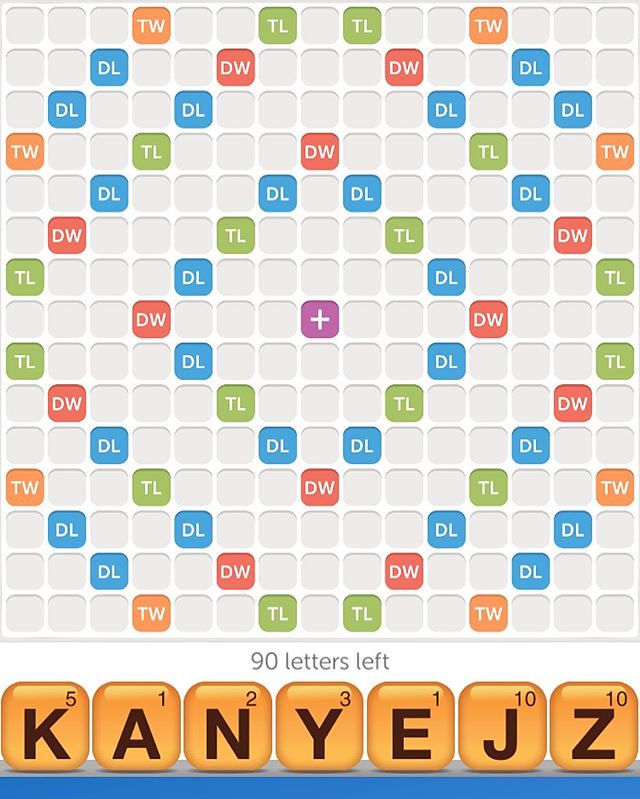This image appears to be a detailed screenshot of a digital Scrabble game, possibly played on a computer or smart device. The board, which takes up roughly 80% of the image, consists of a 20x20 grid of squares, some of which are color-coded in shades of orange, blue, red, green, and purple forming a diamond pattern. The center of the board features a distinctive purple plus sign. Each colored square is marked with abbreviations such as TL (Triple Letter), DL (Double Letter), DW (Double Word), and TW (Triple Word), indicating their point values.

At the bottom of the screen is a blue shelf displaying the player's current letters, which are K, A, N, Y, E, J, and Z. Directly above the shelf, a label reads "90 letters left" in orange text, indicating the remaining tiles in the game. The board and letters stand out against a background that includes white and gray elements, emphasizing the game's layout and colors. The overall appearance suggests the engaging nature of an online Scrabble match, capturing the interactive essence of the game.